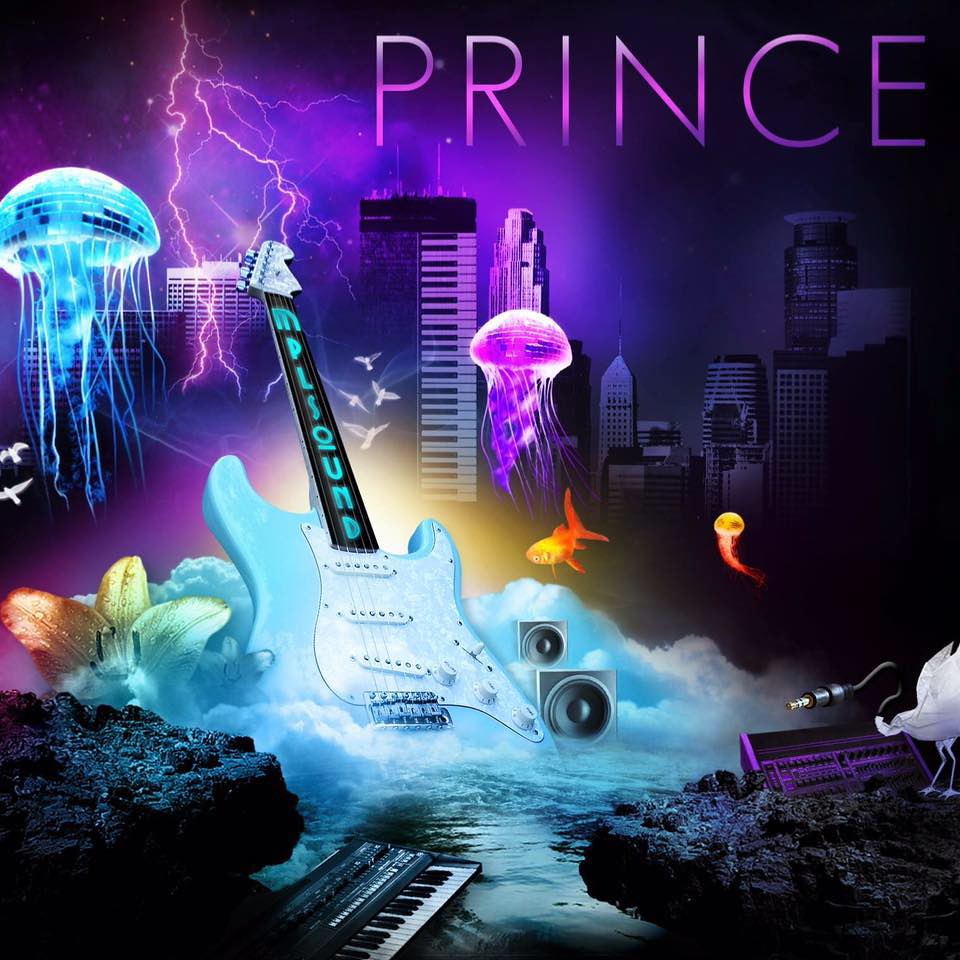This image is a vibrant and detailed digital artwork, resembling a Prince album cover or poster with a purple and blue cloud background. At the top right, the word PRINCE is boldly displayed in all capital letters, blending from light lavender at the top to a deeper, richer purple at the bottom. Below this, a city skyline punctuates the horizon, with piano keys integrated into the buildings.

Dominating the composition are two jellyfish, one blue and one purple, their tops resembling disco balls. The blue jellyfish floats to the left while the purple one hovers centrally. A large light blue and white electric guitar with a black handle extends upward and to the left from the center, with "MPL SOUND" illuminated along its neck. This guitar emerges from smokey clouds at the base, blending into an ocean motif where piano keys can be seen partially submerged.

Enhancing this surreal seascape are goldfish with yellow heads and orange tails, swimming randomly near the ocean waves and dark rocks. White doves soar in the background, adding a serene touch to the energetic scene, while a striking lightning bolt descends from the upper left. 

Overall, this graphic melds elements of music, marine life, and urban landscape into a cohesive and captivating tribute to Prince.